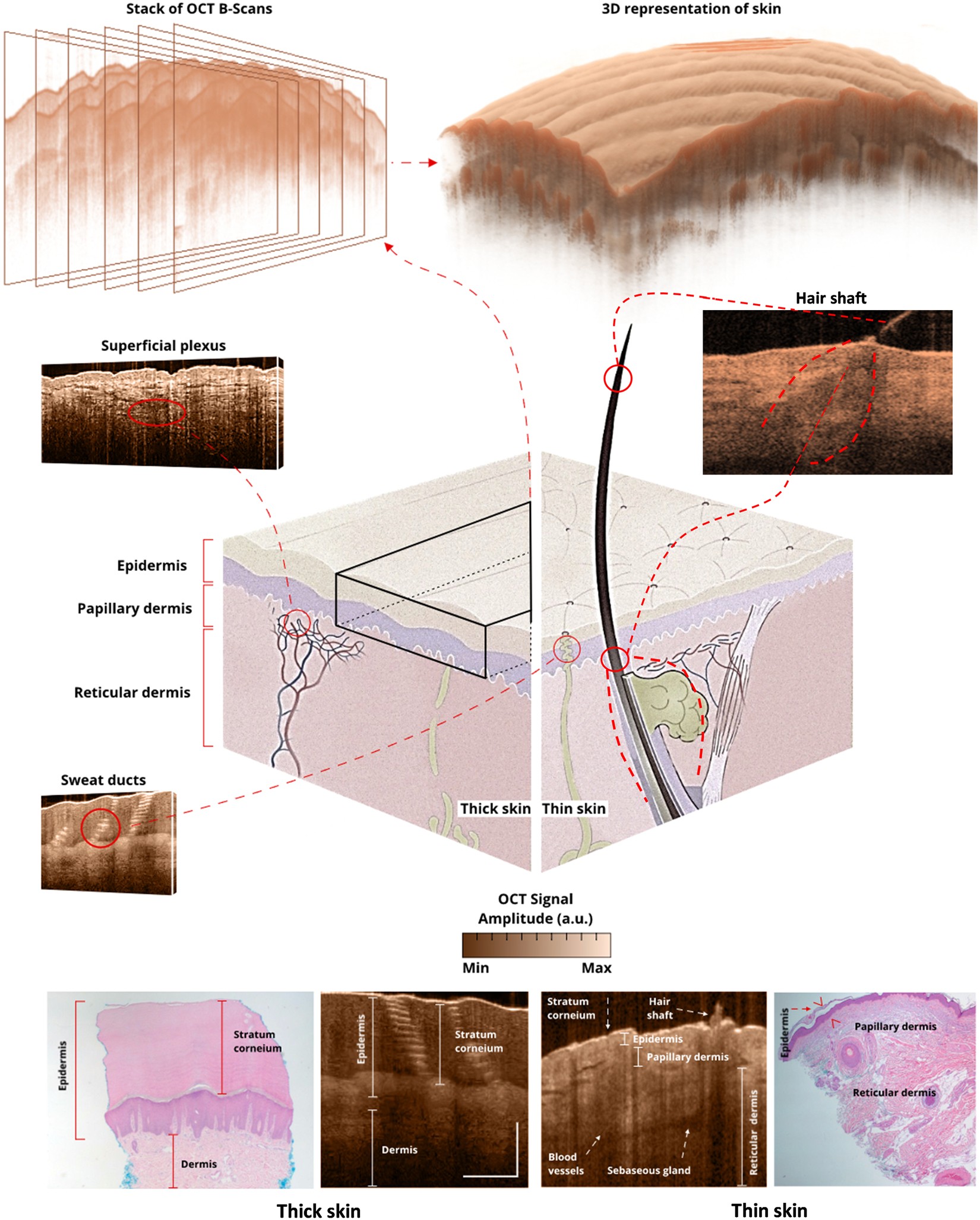This detailed image offers a comprehensive and scientific representation of skin layers and structures. On the left side of the image, a stack of OCT B scans are displayed, providing cross-sectional views of the skin, which are annotated with terms like 'superficial plexus'. On the right side, a 3D representation of skin is presented, highlighting a hair shaft. A central see-through diagram meticulously labels various skin components, including the epidermis, papillary dermis, reticular dermis, capillary dermis, sweat ducts, thick skin, and thin skin. A legend also depicts the OCT signal amplitude from minimum to maximum values. At the bottom part of the image, there are photographs contrasting thick skin and thin skin, showcasing pink structures within the skin layers. The entire layout gives a detailed visualization of the skin's anatomy for scientific or medical analysis.